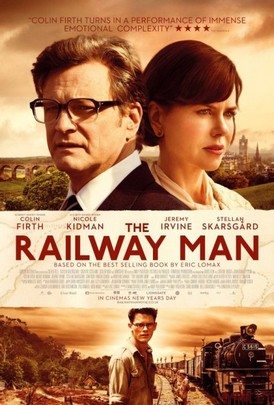The movie poster for "Railway Man" prominently features the title in the center, flanked by names above it: Colin Firth, Nicole Kidman, Jeremy Irvine, and Stella Skarsgård. The top section showcases two main characters: Nicole Kidman, with red hair, facing right in a cream-colored shirt, and Colin Firth, dressed in a dark suit and black glasses, facing left. The background depicts a hazy, brown-clouded sky above a city skyline and bridge. Below the title, text reveals the film is based on the best-selling book by Eric Lomax, interspersed with critical acclaim stating, "Colin Firth turns in a performance of immense emotional complexity," followed by four red stars. The bottom of the poster features a young man standing on train tracks, with a train curving behind him and a man in the background under a similarly brown-clouded sky, framed by hints of a natural landscape. Black text at the very bottom contains credits, though it is too small to read clearly.